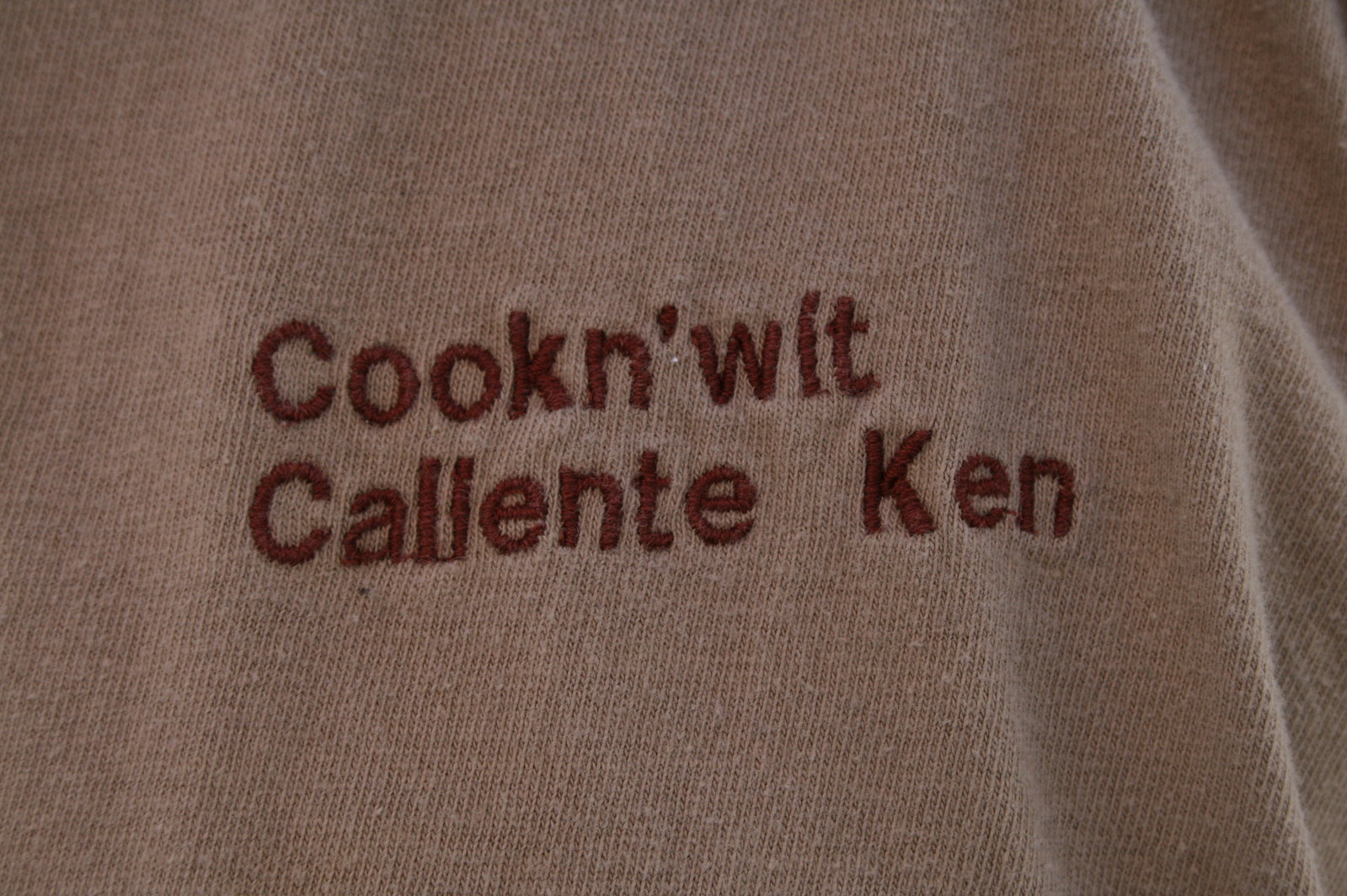This color photograph, oriented horizontally, captures a closeup view of a soft cotton shirt. The fabric, in a light pinkish-brown or beige hue, shows very light pilling. A folded piece of fabric appears on the right-hand side of the image, bathed in light coming from the same direction. Central to the image is an embroidered section of the shirt, with text in a burnt sienna, dark brown color that reads "COOKIN' WIT CALENTE KEN." The embroidery stands out against the light background, showcasing the detailed craftsmanship and texture of the material.